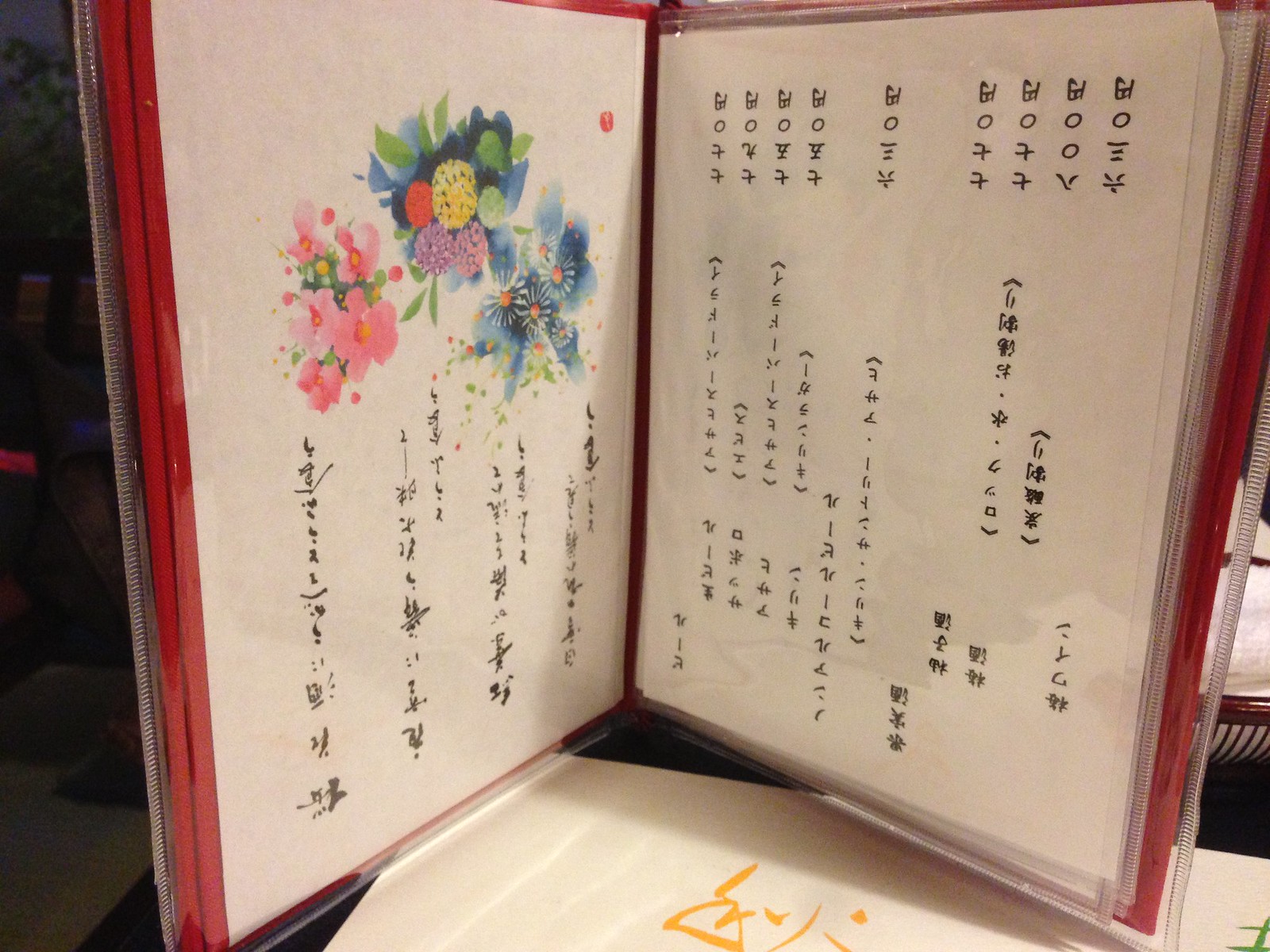The image depicts a photograph taken indoors of a small, open red binder resting on a dark black table. The binder contains plastic sleeves protecting the pages within. On the left-hand page, intricately hand-drawn Chinese characters are flanked by decorative floral illustrations. There are three distinct floral designs featured at the top: a bouquet of pink and light pink flowers with green leaves, a bundle including yellow, green, purple, and red elements, and a collection of blue sunflowers. The right-hand page primarily showcases handwritten Chinese characters arranged in vertical columns, perhaps listing items with prices. A white piece of paper adorned with yellow designs peeks out from beneath the binder, which sits slightly askew, revealing a hint of the space surrounding the scene.